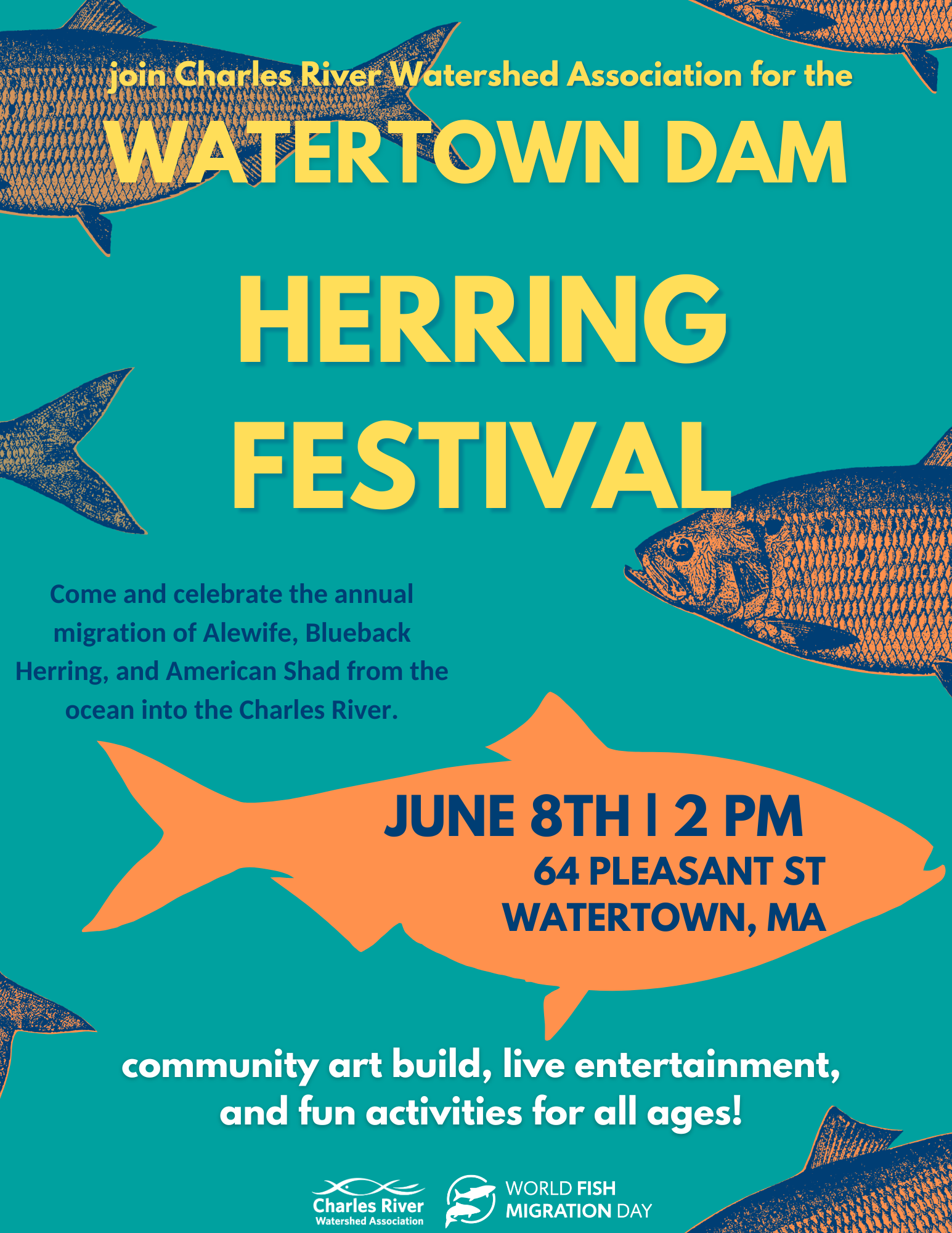The color image is a vibrant and festive advertisement for the Watertown Dam Herring Festival, set against an aqua blue background. This visually engaging poster features partial illustrations of herring, artfully cropped on either side to frame the central information. The main text, highlighted in bold yellow font, invites viewers to "Join Charles River Watershed Association for the Watertown Dam Herring Festival." 

Beneath this, in smaller blue type, it details the event's focus: "Come and celebrate the annual migration of alewife, blueback herring, and American shad from the ocean into the Charles River." Adding a splash of contrast, an orange silhouette of a fish adorns the bottom portion of the poster, with the essential event details inscribed in dark blue text within the silhouette: "June 8, 2 p.m., 64 Pleasant Street, Watertown, Massachusetts." Finally, the poster caps off with a promise of engaging activities, noted in white text at the very bottom: "Community Art Build, live entertainment and fun activities for all ages."